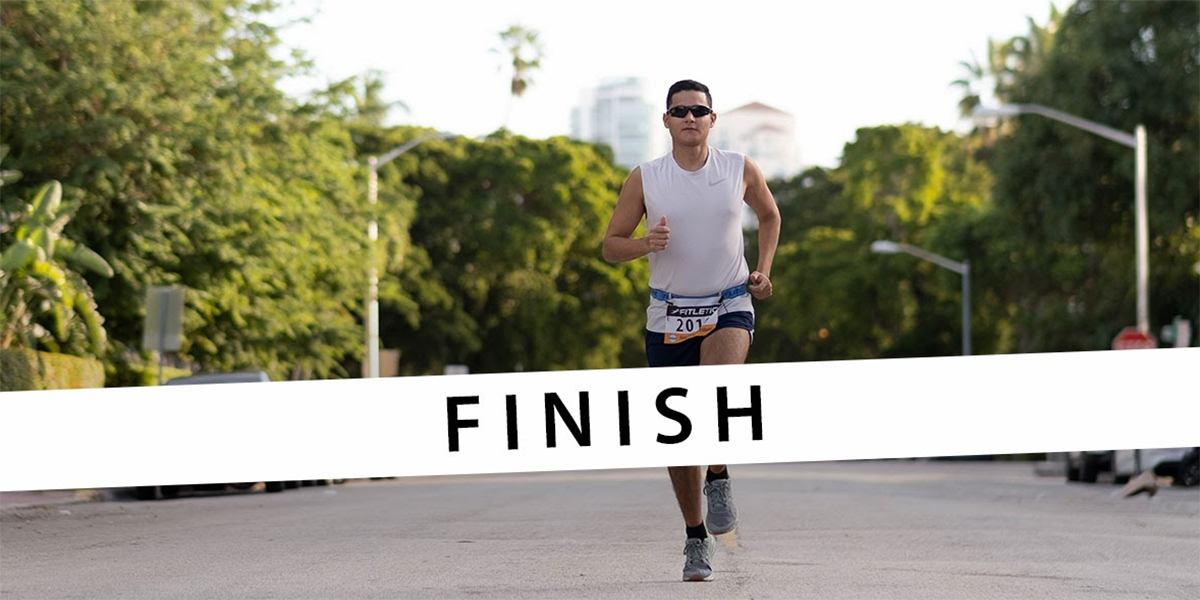A solitary Caucasian male with short, dark hair and black sunglasses is running a marathon on an asphalt street lined with green trees and light poles. He's clad in a white sleeveless t-shirt emblazoned with a gray Nike logo, blue and white shorts, black socks, and gray sneakers. Around his waist, a race number "201" is visibly attached. He approaches a diagonally positioned, likely photoshopped, white banner with "FINISH" written in bold black letters across it. The street appears deserted, with some distant cars and buildings visible far off in the background under a shiny sky with the sun gleaming down.